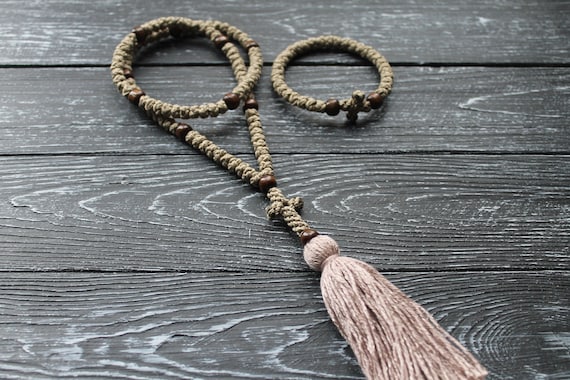The image shows a set of handmade decorative bracelets arranged on wide-planked, dark gray wooden floors with white accents. The bracelets, made of medium brown woven twine, include intricate details and crosses fashioned from the same material. One bracelet, positioned to the right, features a meticulously crafted cross at the top. Another bracelet displays small dark brown beads along its sides, and a larger bracelet beneath both boasts another cross with a long, beige tassel extending from it. The lighting and quality of the photograph are commendable, giving it a professional yet slightly imperfect appearance, and the overall setting is characterized by neutral sandy and brown tones without any text.